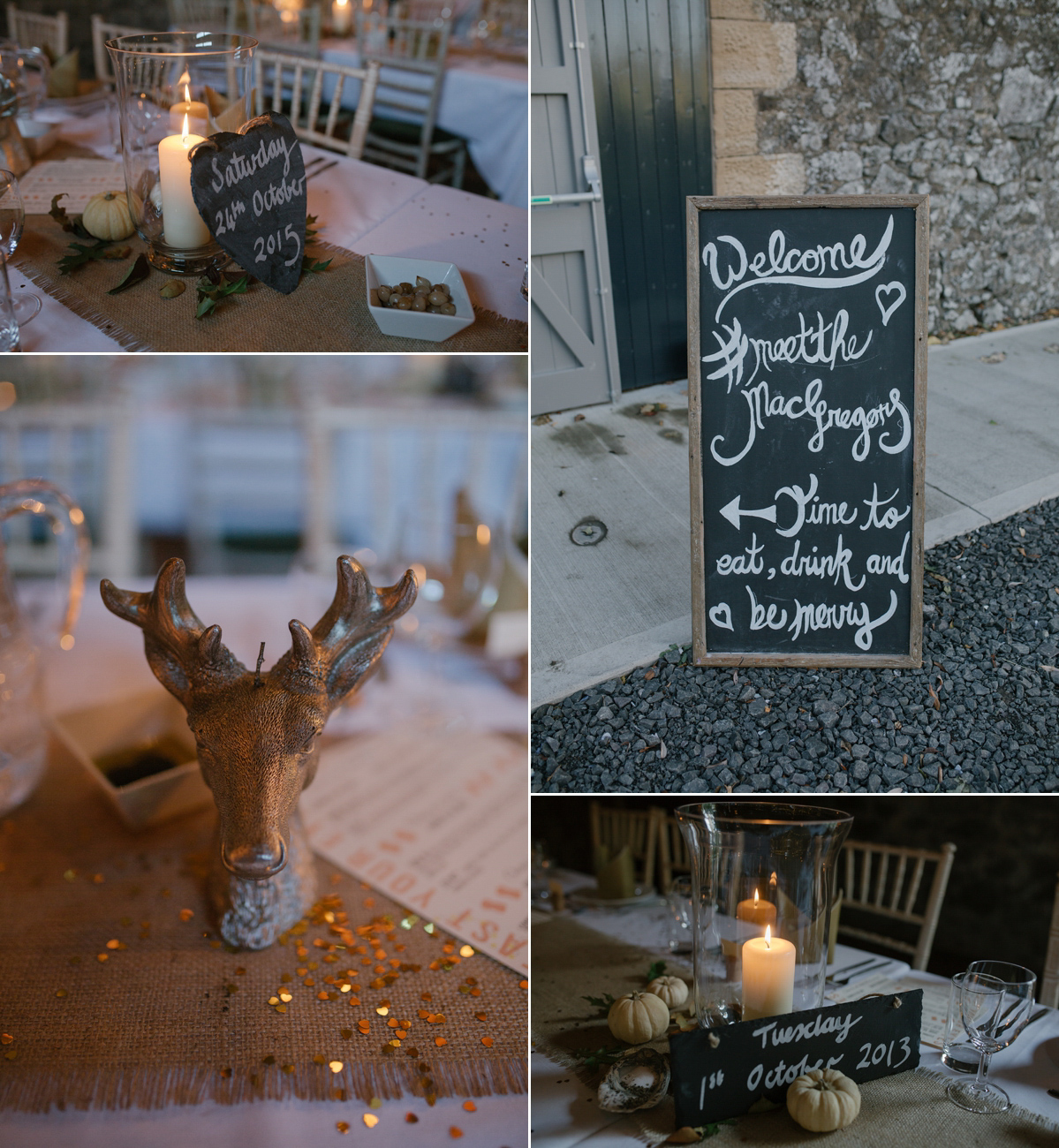This image is a vertical collage comprising four photographs that collectively depict a rustic fall-themed gathering setup with a mix of indoor and outdoor elements. In the top left corner, a tastefully decorated table with a white tablecloth is enhanced by a brown linen runner. The table settings include plates, cutlery, a burning candle, a white pumpkin, and a distinctive black heart-shaped chalkboard that reads "Saturday, 24th October 2015." The bottom left photo focuses on a bronze-colored deer head sculpture placed on a burlap placemat, adding a touch of glitter and charm to the arrangement. The top right photo shifts the scene outside, showing a chalkboard easel on gravel next to a walkway and partial door. The chalkboard welcomes guests with the message: "Welcome, Meet the McGregors, Time to Eat, Drink, and Be Merry," complete with a cutesy heart symbol. Finally, in the bottom right photo, the same fall-themed table is revisited, this time with additional white pumpkins surrounding a candle. A rectangular chalkboard on the table now reads "Tuesday, 1st October 2013," adding to the collage's nostalgic and celebratory ambience.